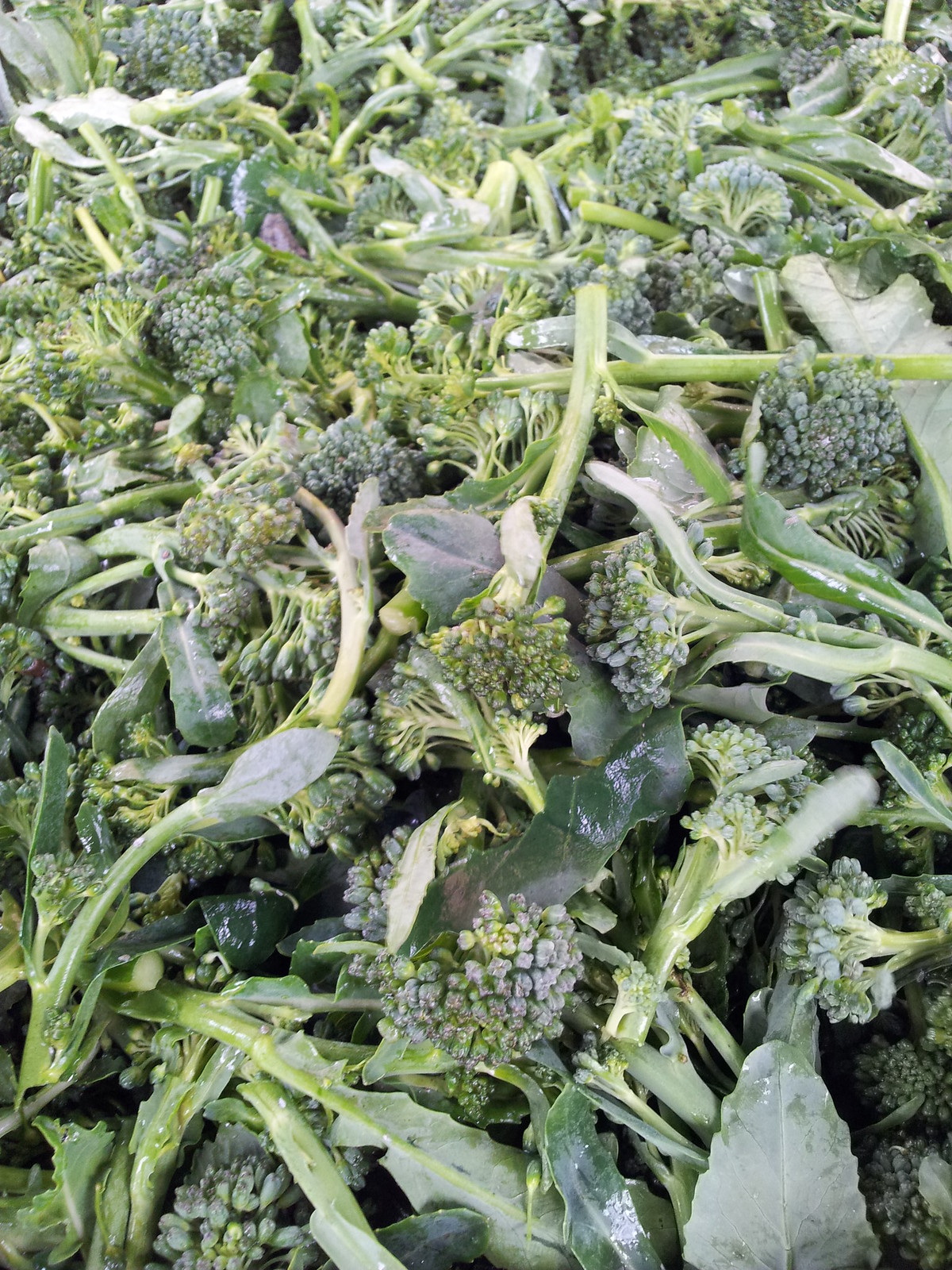This detailed caption combines and clarifies the repeated elements from each description:

---

The image is a close-up, portrait-oriented photograph entirely filled with freshly harvested broccolini. The broccolini is piled chaotically, with no specific arrangement, as if it has been dumped onto a surface, which is not visible in the picture. The pile consists of thin, light green stems topped with puffy green crowns, and interspersed are broad, dark green leaves with prominent veins. The image showcases varying shades of green—light, dark, and frosted—giving a sense of the freshness and diversity in color. There are hints of purple hues on some leaves, suggesting a natural variation often found in broccoli. The broccolini appears clean and washed, though some pieces still carry bits of dirt, reinforcing its freshly harvested nature. The photograph likely depicts the produce ready for preparation or sale, capturing a detailed and vibrant snapshot of the vegetable's different parts—stems, leaves, and florets.